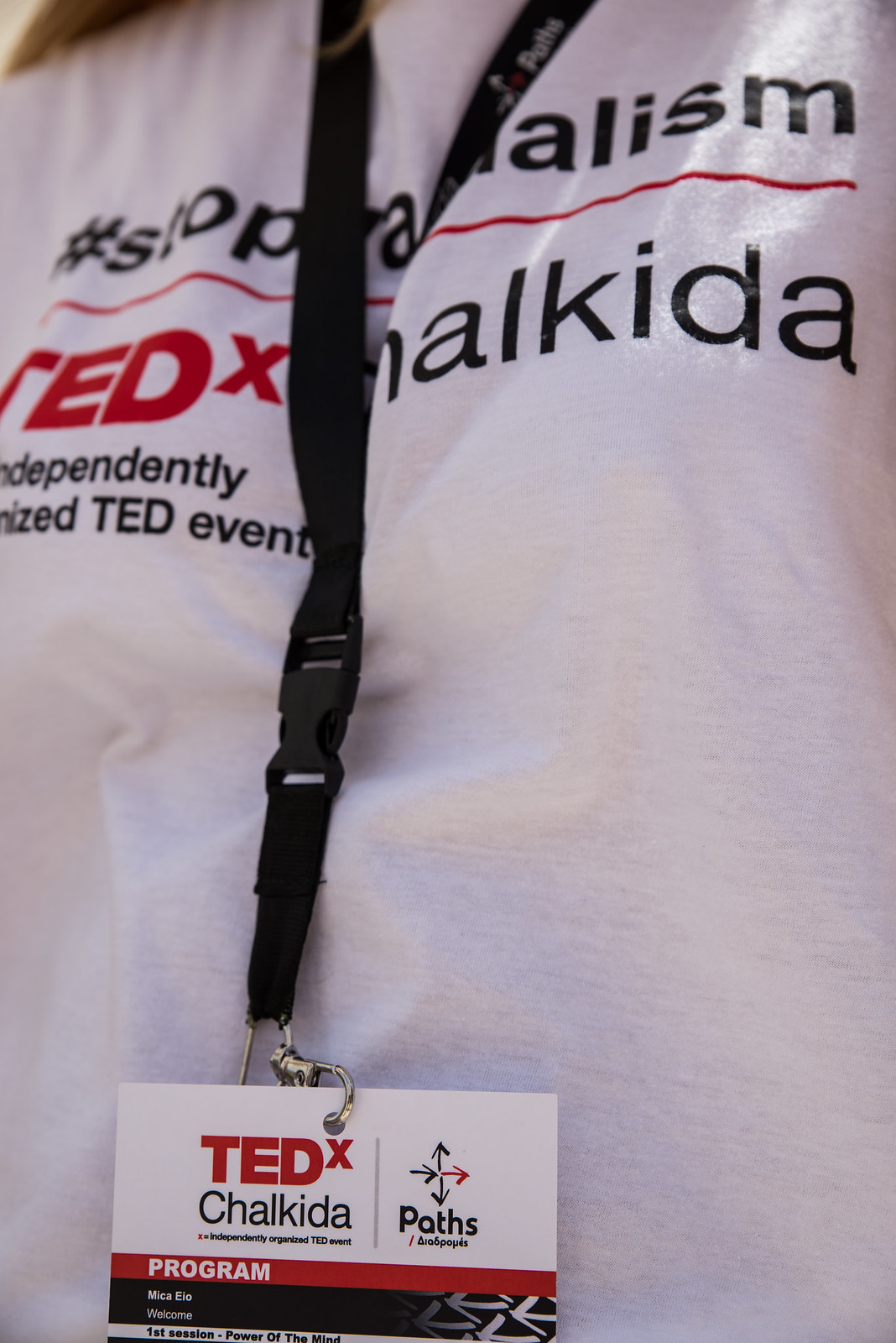The image shows a cropped view of the front of a wrinkled white t-shirt with black and red text. The person wearing this t-shirt also has a black lanyard around their neck, from which an ID badge is hanging. The badge displays "TEDxChalkida," indicating it is an independently organized TED event. The shirt partially hides a hashtag slogan, likely reading "#StopCapitalism," although the folds obscure the exact wording. Below the disputed hashtag, the shirt clearly shows "TEDx" in bold red letters, followed by "Chalkida" in thin black text, and the phrase "independently organized TED event." The ID badge also mentions details about the event's program, specifying a session titled "Power of the Mind" and the name "Miko Io." The image seems to focus more on the attire and badge rather than the person, whose face isn't visible, but appears to suggest a woman based on the outline visible through the shirt.